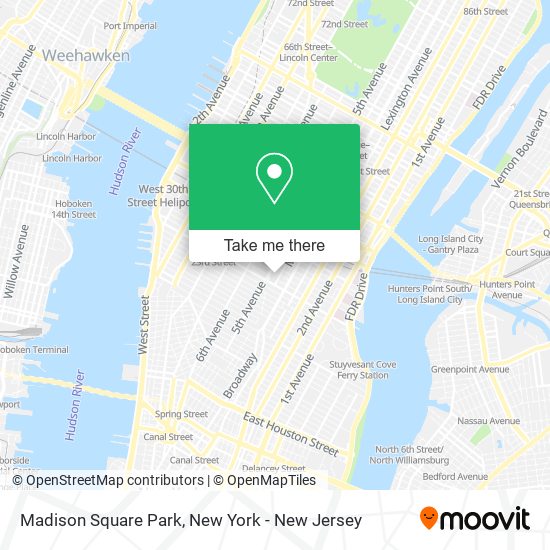This image appears to be a screenshot from Google Maps. The background consists of a detailed map with various streets labeled in dark gray text. In the center background, there is a piece of land connected by a thin horizontal yellow line, presumably a bridge. On either side of the map, long, vertical blue lakes are visible.

Dominating the center of the image is a white rectangular box containing another image, likely a nighttime photograph of a park in New York City. This park is characterized by leafless trees bathed in yellow light, creating a moody, dark atmosphere. In the background of this inset image, some illuminated buildings can be seen. Street lamps contribute to the overall glow of the scene.

In the bottom right corner of the image, black text in lowercase spells out "moovit" (m-o-o-v-i-t), accompanied by an orange GPS symbol with a black smiley face at its center. On the bottom left corner, there is black text that reads "Madison Square Park New York - New Jersey" in capital letters. Inside the white box showcasing the city view, blue text says "take me there."